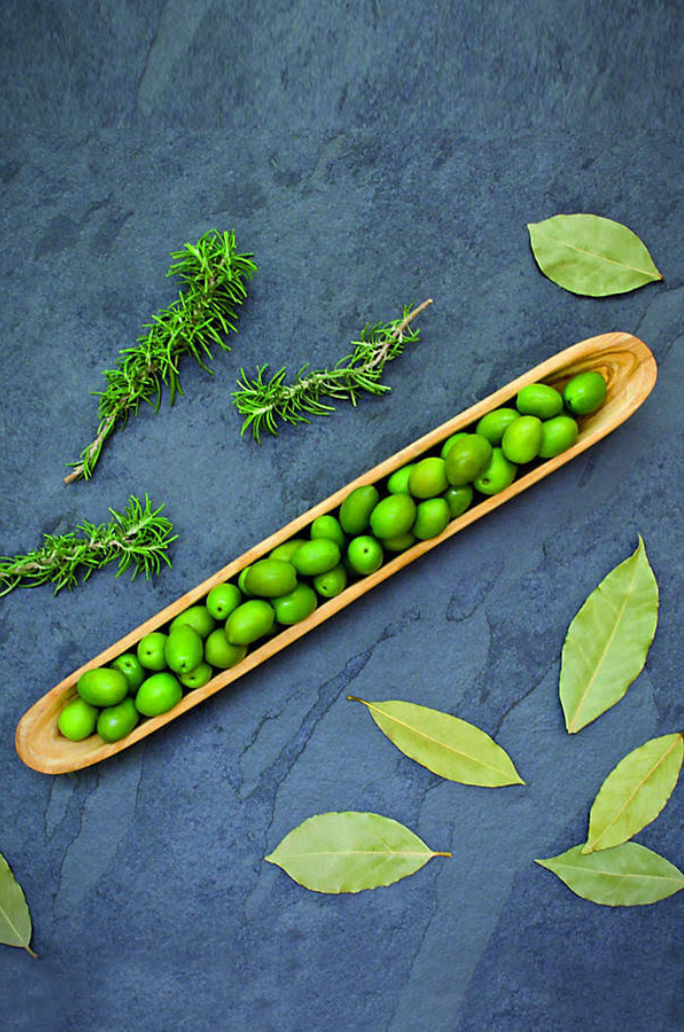This is a top-view photograph capturing a detailed scene on a dark stone or marble surface. At the center, there is a long, oblong-shaped wooden bowl filled with bright green, oval-shaped fruits that resemble edamame beans or green olives. The fruits have small holes at the ends, suggesting they were freshly picked. The wooden bowl is placed diagonally across the image. Surrounding the tray are various herbs; at the top, three sprigs of rosemary lay vertically, while to the top right of the bowl, a single green bay leaf is visible. Additionally, five more bay leaves are sprinkled around the bottom of the bowl. The overall composition and color contrast between the bright green fruits and herbs against the dark stone surface make the image visually striking.